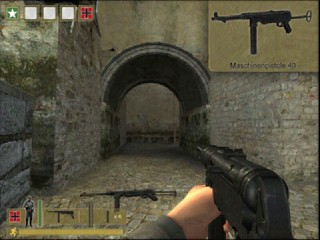In this image, a computer screen displays an intense moment from a first-person shooter game. At the forefront, a pale pink hand grips a substantial black machine gun, aiming directly at a shadowy, arched tunnel in the background. The tunnel is constructed from grey stone, some of which is overgrown with green moss, conveying an aged and weathered look. The stone grey flooring stretches out towards the tunnel, which is partially topped with patches of grey stucco above its entrance, adding to the dilapidated ambiance.

In the upper right-hand corner of the screen, there is an icon depicting a long black weapon, identifying the player's current armament. On the left side of the screen, a star, three small squares, and a red cross serve as part of the in-game interface, possibly indicating objectives, resources, or health status. The bottom left corner features additional icons representing a character and various weapons, giving further information pertinent to the gameplay experience.